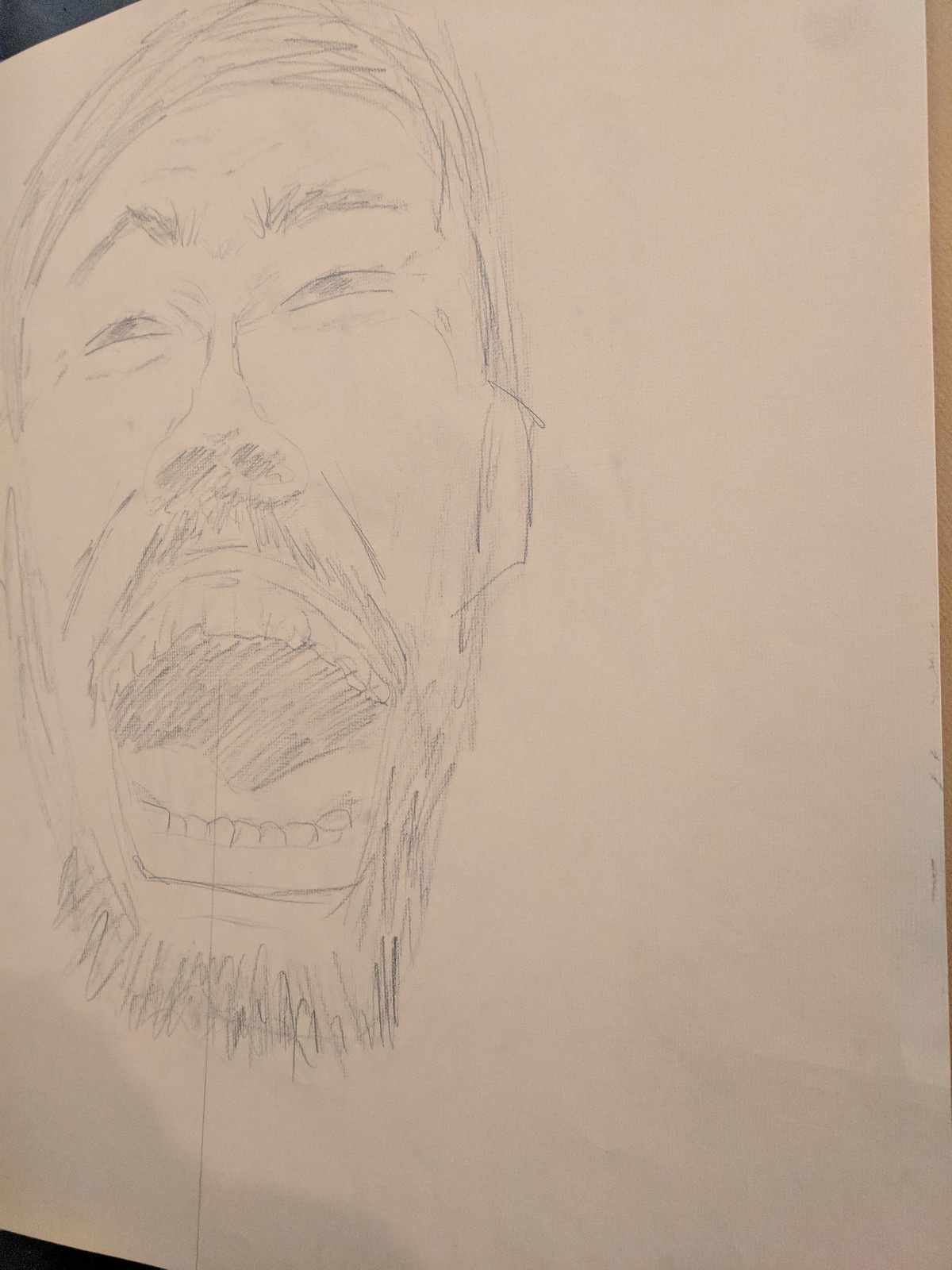This detailed photograph showcases a hand-drawn portrait on a standard white sheet of printer paper. The drawing appears to be executed primarily with pencil, possibly augmented with pen for finer details. Captured at a slight angle, the image shows some skewness, adding a dynamic perspective to the artwork. The portrait features a male figure with short hair and noticeable facial hair, including a mustache and beard. His mouth is wide open, revealing his tongue and teeth, indicative of a shouting or screaming expression. The subject's slightly bushy eyebrows are arched, enhancing the intense emotion conveyed, perhaps anger or distress. The artist's rendering suggests the figure might be of Asian descent, adding another layer of depth to the compelling representation.